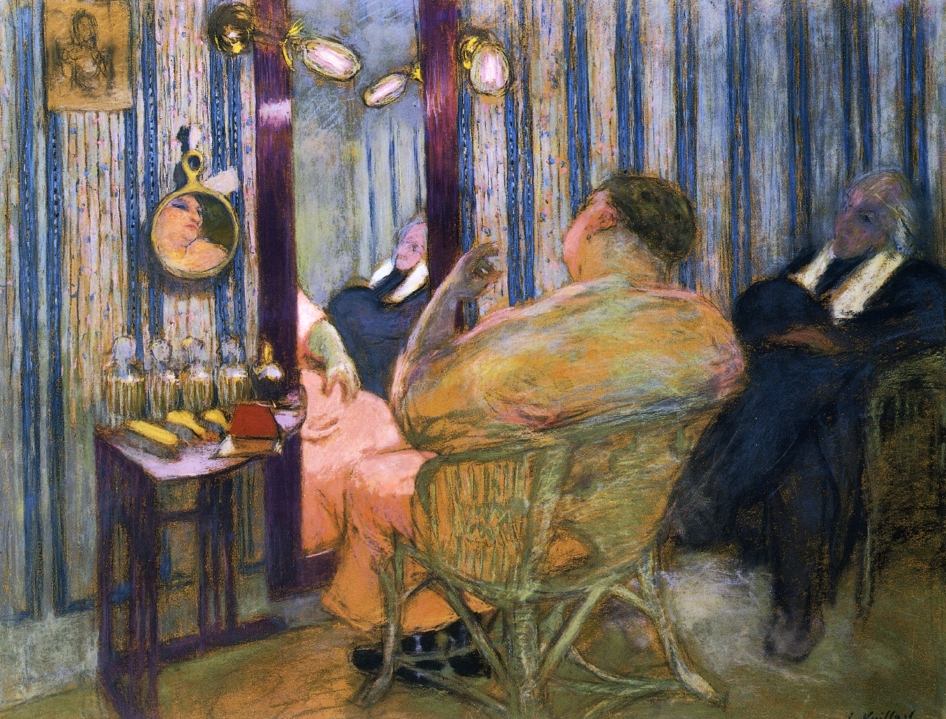The painting depicts an indoor scene featuring two individuals seated in a room with elaborate details. At the center, a rather large individual, possibly a man, is seated in a thin, wicker-style wooden chair, wearing pink clothes and looking directly at a full-length mirror with a purple border. The person, of Caucasian descent with dark blue or purple eyeshadow, thin lips, and a straight hooked nose, focuses intently on their reflection. The mirror, adorned with lights at the top, is mounted on a wall decorated with blue and white vertical stripes interspersed with rectangular patterns and small blue dots. 

Adjacent to this person on the right side of the painting sits another individual, who appears older with dark brown skin and white hair on the sides. This person is attired in dark clothing that resembles either a black coat or judge's robe, contrasted by a white collar or scarf, exuding an air of formality. They sit cross-legged, with their hands resting on their lap, seemingly engaged in a conversation, though their gaze is directed towards the first individual rather than the mirror.

To the left of the main figure is a small dressing table cluttered with items, including a book, brushes, bottles, and various other objects. Above this table hangs a smaller, circular mirror, positioned upside down, which also captures the reflection of the main individual. In the upper left-hand corner of the wall, a sketch of a person can be seen, adding another layer of depth to the intricate setting.

The ground of the room is brown, complementing the chairs the individuals are seated on, creating a cohesive color palette that enhances the overall composition of the painting.